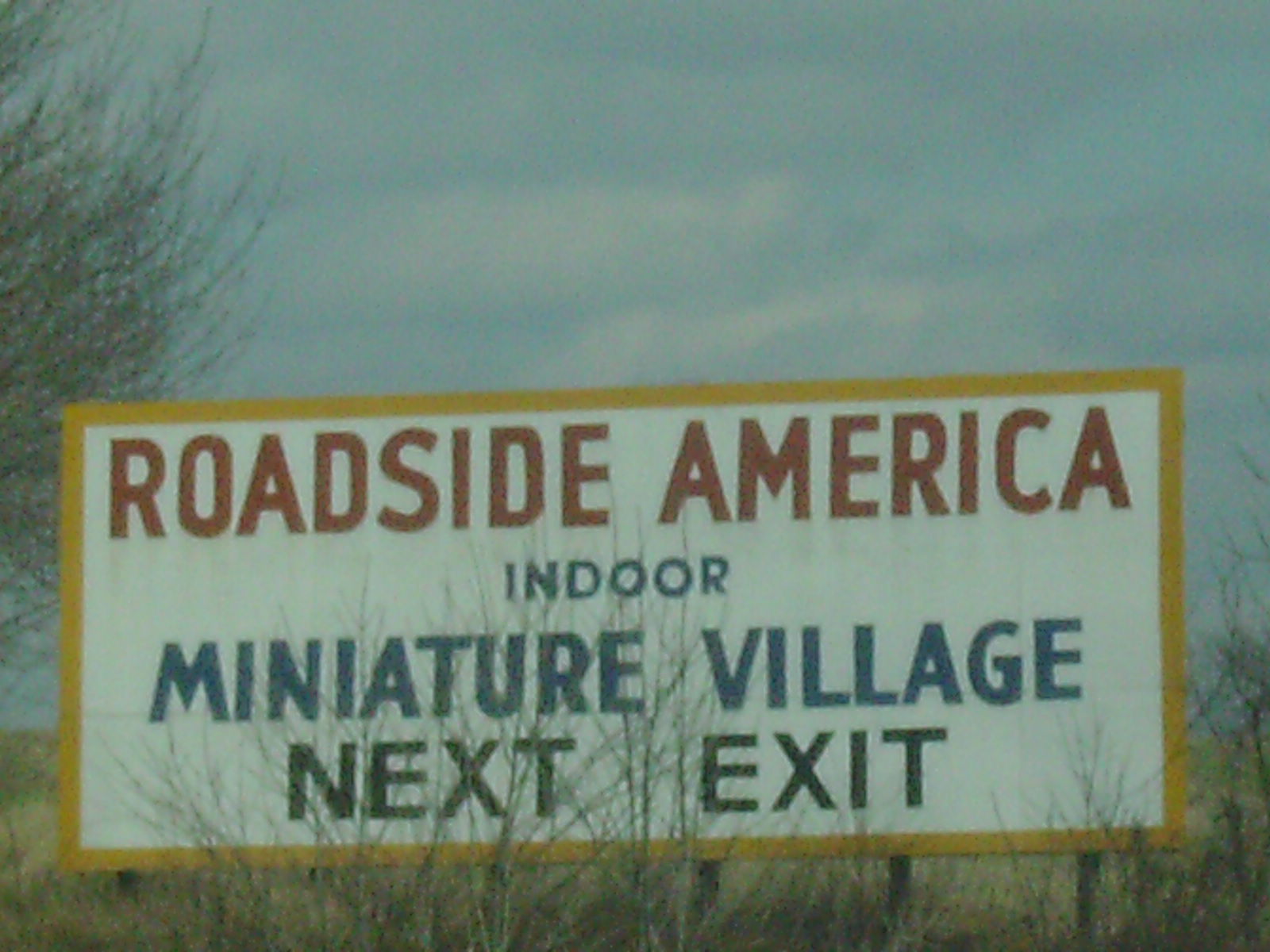A large billboard stands prominently against a bright blue sky dotted with clouds, advertising "Roadside America," an indoor miniature village. The billboard features bold white, red, black, and blue letters, making it highly visible to passersby. Supported by sturdy, round metal structures, the base of the billboard is partially obscured by overgrown grass and bushes, blending it into the natural surroundings. Adjacent to the sign is a tree with sparse leaves, enhancing the rural, countryside ambiance of the scene. The overall setting is characterized by wild grass and a tranquil, pastoral landscape.